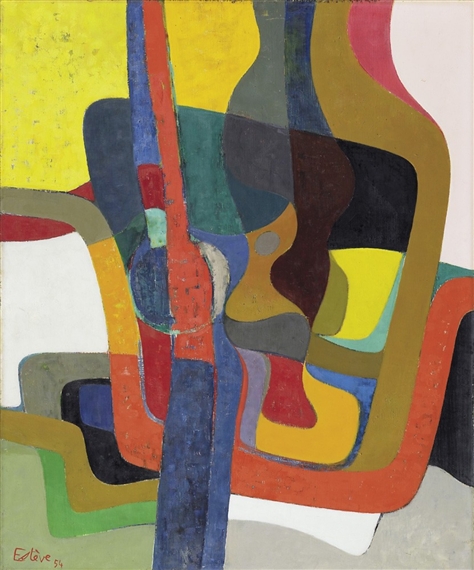The abstract painting vividly plays with a multitude of colors and shapes, creating a chaotic yet intriguing scene. Prominently featuring a signature in the bottom left corner written in red ink, beginning with 'E' and ending in '54', the artwork is notably complex and mysterious. The upper left corner is dominated by a bright blotch of yellow, transitioning into thick red and blue strings that extend downward. These strings merge into a ball at the center, where the red string turns blue and continues its descent.

The composition is further enriched by a warped square in the background, displaying a gradient from blue, black, yellow, orange, and a touch of teal in various corners. To the top right, it appears as if water is streaming down, painted in shades of brown and pink, pooling onto a gray ground. The entire scene seems to rest on a wrinkled, arching carpet, casting a black shadow on the bottom right.

Blended into this design, there's a suggestion of a face in the middle section. Interpreted by some, this face has a blue eye, a brown nose, blue hair, and a red section below resembling a tongue, with black strokes hinting at hair. Vivid lines and stripes in red, blue, brown, yellow, green, and purple intersect around this symbolic visage, adding to the painting's enigmatic allure.